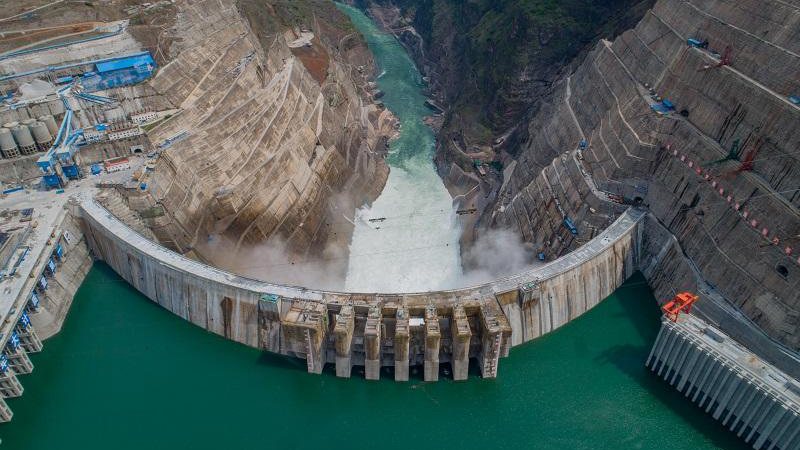An aerial photograph showcases a massive, curved dam nestled within a steep rock canyon, reminiscent of a waterfall's summit. The dam, positioned centrally, stretches from left to right in a half-moon shape, effectively halting the river's flow far below and creating an expansive, green-hued artificial lake behind it. On the right, the rugged, high mountain slopes add dramatic framing to the scene, likely marking the river's ancient pathway. Notable construction activity can be observed on the left side of the dam, featuring bluish structures and cranes. The sheer rock faces exhibit varying levels, resembling pathways that seem to beckon one to explore the precipitous terrain. The colors in the image range from blue-green to lighter blue-green waters, set against a backdrop of tannish-gray, gray, and hints of red from the canyon walls. The absence of text in the image invites a pure focus on the intricate and captivating details of this remarkable landscape.